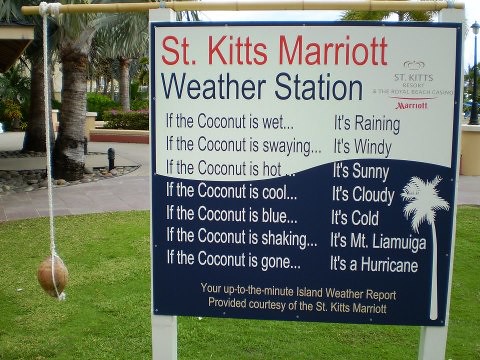This image features a sign displayed at the St. Kitts Marriott resort, detailed in a playful manner to entertain guests. The sign is affixed to two white wooden poles planted in a short, green grassy area, with a brick walkway and palm trees visible behind it. The sign itself is divided into two halves—a white top and a blue bottom. At the very top in bold red letters, it reads "St. Kitts Marriott," followed by "Weather Station" in blue. 

The most eye-catching element of the sign is a small brown coconut hanging from a rope attached to a bamboo shoot at the top of the sign. Below this, the sign humorously provides weather predictions based on the coconut's condition: "If the coconut is wet, it's raining. If the coconut is swaying, it's windy. If the coconut is hot, it's sunny. If the coconut is cool, it's cloudy. If the coconut is blue, it's cold. If the coconut is shaking, it's Mount Liamuiga. If the coconut is gone, it's a hurricane." There is also a small palm tree illustration and the St. Kitts Marriott logo on the top right corner of the sign. At the bottom, it concludes with "You're up to the minute island weather report provided courtesy of the St. Kitts Marriott." This charming display is just one of the amusing touches designed to enhance the tropical experience for resort visitors.